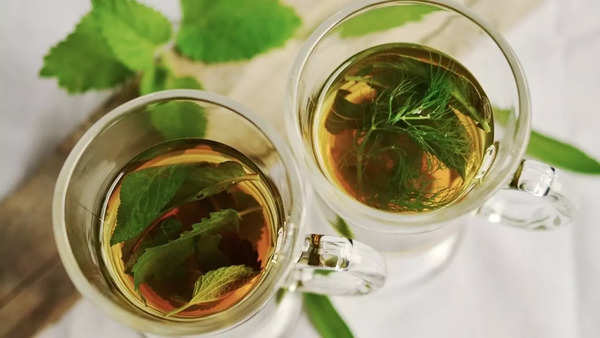This is a close-up, top-down photograph of two clear glass mugs of herbal tea, placed on a white cloth-covered table. Both mugs have right-side handles. The liquid inside them is a light brownish-orange color, likely tea, with various herbs floating or sunk to the bottom. The left-hand mug contains four dark green mint leaves floating on the surface. The right-hand mug includes both green mint leaves and finer green herbs resembling dill, some of which are sinking to the bottom. Between the two mugs and reflected on their surfaces, additional mint leaves are visible. To the right of the right-hand mug, a single leaf rests on the white cloth. Behind the mugs, to the left, a portion of brown fabric is faintly discernible against an otherwise blurred background.